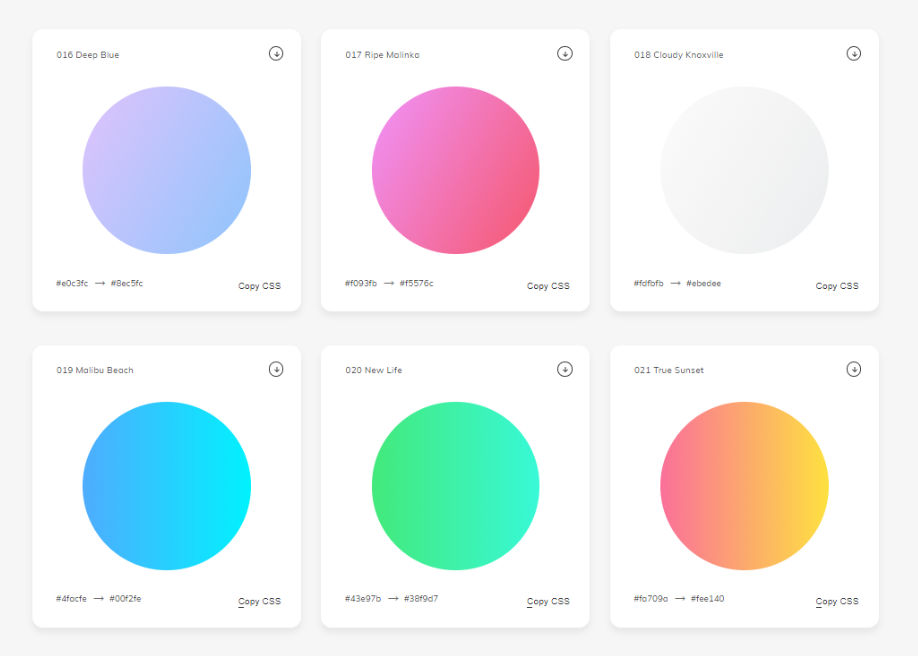The image is a square that contains six smaller squares arranged in two rows of three. Each smaller square showcases a color swatch, including its name, a sample circle of the color, as well as corresponding color codes, and an option to copy CSS. 

- **Top Row:**
  1. **016 Deep Blue**: 
     - Color Sample: Blue
     - Hex Codes: #E0C3FC ➡️ #BEC5FC
     - Option: Copy CSS
  2. **017 Ripe Malinka**:
     - Color Sample: Hot Pink
     - Hex Codes: #F093FB ➡️ #F5576C
     - Option: Copy CSS
  3. **018 Cloudy Knoxville**:
     - Color Sample: Gray
     - Hex Codes: #FDFAFA ➡️ #EBEDEE
     - Option: Copy CSS

- **Bottom Row:**
  4. **019 Malibu Beach**:
     - Color Sample: Teal/Turquoise
     - Hex Codes: #4FACFE ➡️ #00F2FE
     - Option: Copy CSS
  5. **020 New Life**:
     - Color Sample: Green
     - Hex Codes: #43E97B ➡️ #38F9D7
     - Option: Copy CSS
  6. **021 True Sunset**:
     - Color Sample: Gradient from pink to orange
     - Hex Codes: #FA709C ➡️ #FEE140
     - Option: Copy CSS